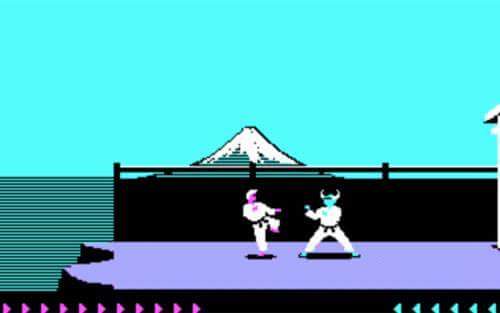The image depicts a vibrant scene from a fighting video game, showcasing two kung-fu fighters engaged in combat. Both fighters are attired in traditional white karate outfits with black belts. The fighter on the left boasts a pink hue for their head, hands, and feet, paired with white hair, and is poised with their left leg raised, as if ready to kick. The opponent, on the right, has a striking blue complexion on their face, hands, and feet, and sports prominent devil-like horns on their head. This fighter appears to be preparing to throw a punch with their legs spread apart.

The battleground features a purple platform with black sides, suggesting a daunting cliff drop at its rugged edge. Behind the fighters stands a majestic mountain, reminiscent of Kilimanjaro, blanketed with patches of snow. A solid black fence demarcates the fighters' area from the picturesque, yet ominous, mountain backdrop. The bright blue sky above and the subtle blue-toned water to the left side, represented by thin dark blue lines, enhance the overall vividness of the scene, merging seamlessly into the teal blue-green horizon.